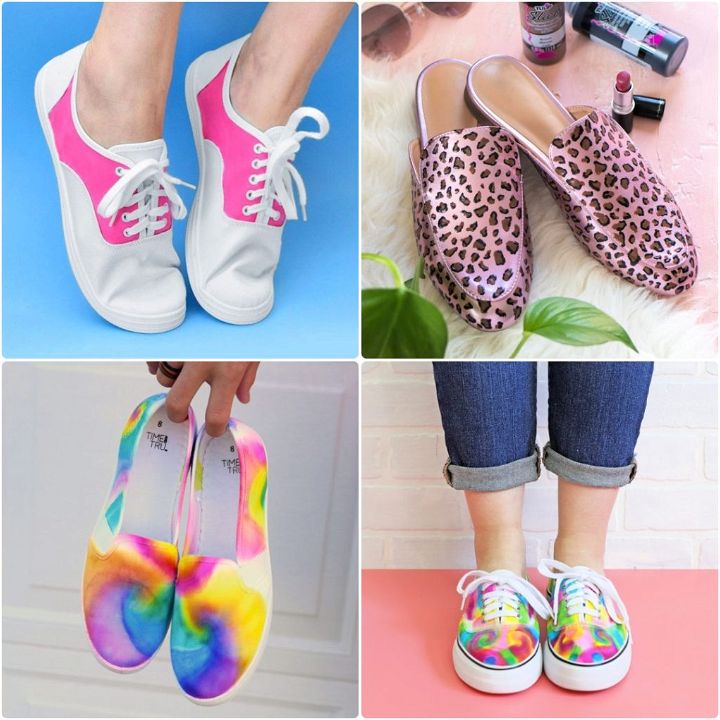This is a photo grid consisting of four equally-sized images, divided two by two, each showcasing a different pair of fashionable shoes. 

In the top left quadrant, the photo depicts a woman standing on her tiptoes against a blue background, wearing white low-top shoes with pink details akin to Vans or Converse styles. 

The top right image features a pair of shiny pink leopard print slip-on shoes placed on a white fur carpet, surrounded by makeup, hairspray, and sunglasses, giving a glamorous vibe.

In the bottom left quadrant, a pair of rainbow tie-dye slip-on shoes, resembling knockoff Vans, are held up against a white door or cabinet, with only the holder’s fingers visible.

The bottom right photo shows a person, dressed in blue jeans, standing on a pink floor with a white brick wall behind them, wearing rainbow tie-dye low-top, lace-up shoes. 

The background elements and diverse shoe designs create a dynamic and colorful display, suggesting that this image is likely part of an advertisement.